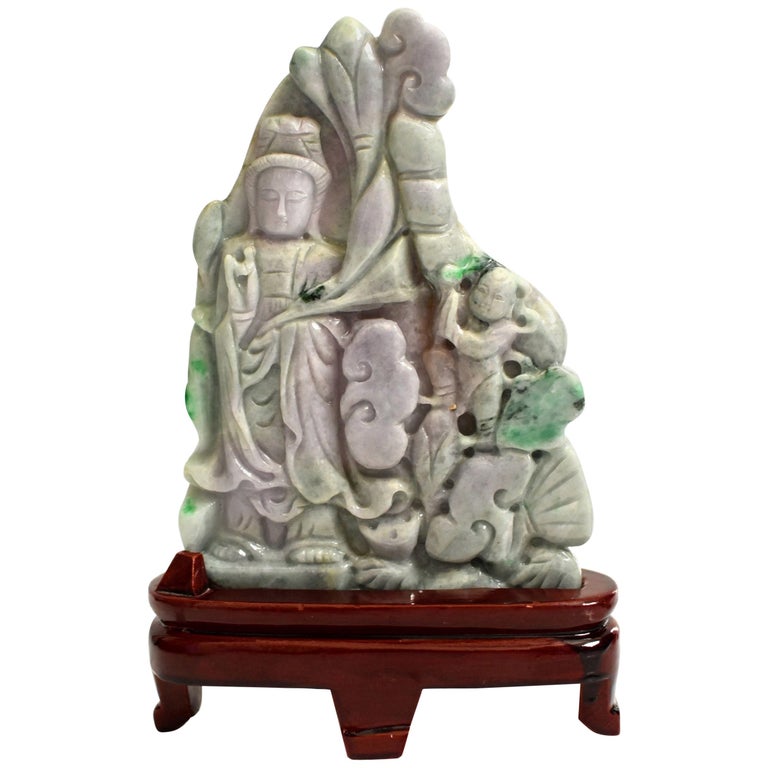The image depicts a finely polished stone carving, likely made of jade due to its green, somewhat translucent appearance. This ancient Chinese artifact features an intricate scene of a Buddhist deity on the left and a child on the right, seemingly traveling amidst misty clouds or sacred trees. The stone is a mix of grey and green hues, with noticeable transparency, enhancing its detailed craftsmanship. The sculpture is prominently positioned in the center of a dark walnut-colored wooden stand, which has a glossy finish and rests on three legs. Surrounding the artifact is a stark, empty white background, drawing complete focus to the delicate and elaborate carvings of the ancient piece.